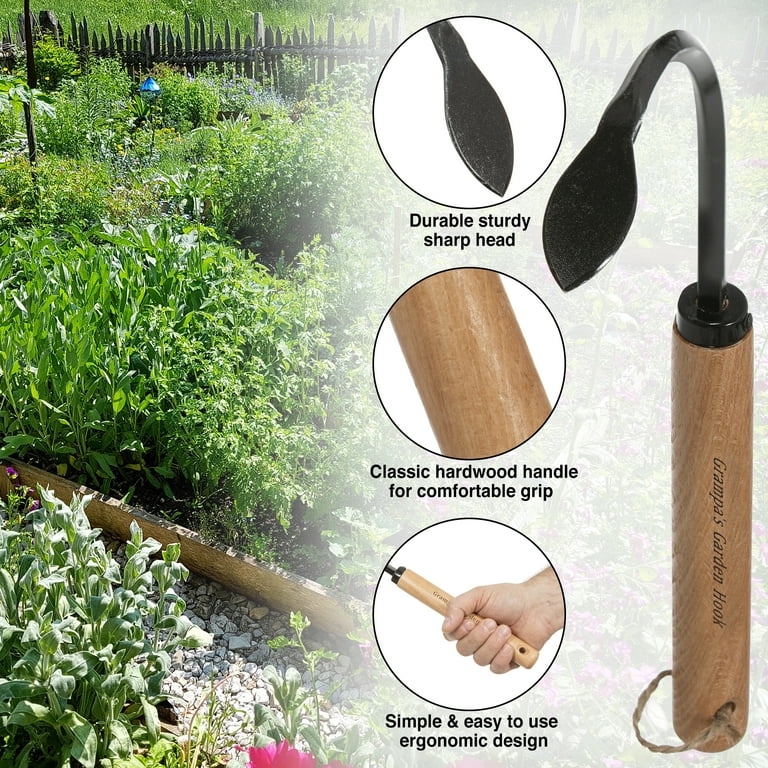The photograph appears to be an advertisement for a gardening tool, distinctly illustrating its design and features. On the left side of the image, there's a vibrant garden showcasing an array of bright green leaves and clearly organized rows, topped with a pointed wooden fence visible at the top edge of the frame. To the right, a white gradient overlays part of the garden, through which a detailed diagram of the tool is visible. The tool itself, positioned vertically on the far right, features a wooden handle engraved with the text "Grandpa's Garden Hook" in black italicized font, and a black metal hook with a leaf-shaped tip that curves to the left. Beside the tool, three white circles with black outlines highlight its features: a close-up of the leaf-shaped tip labeled "durable, sturdy, sharp head," a detail of the wooden handle labeled "classic hardwood handle for comfortable grip," and an image of a hand holding the tool labeled "simple and easy to use ergonomic design." This comprehensive visual and textual information effectively advertises the garden hook, emphasizing its durability, ergonomic design, and comfortable grip.